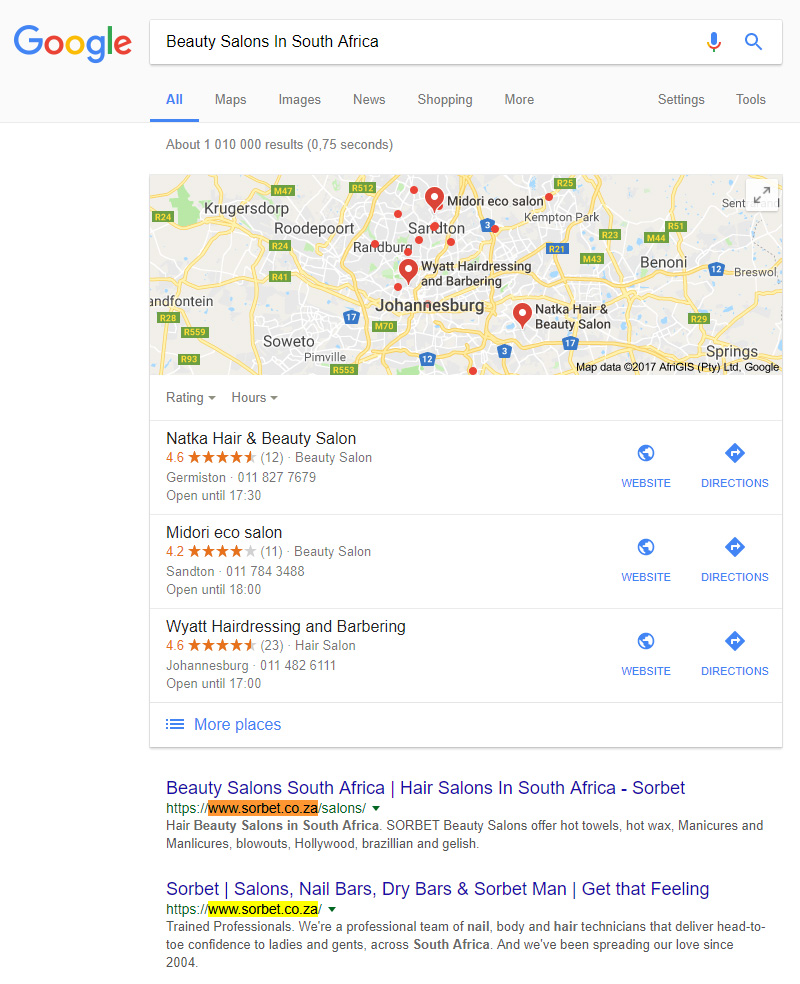The image shows a detailed Google search results page for beauty salons in South Africa, specifically highlighting several options in Johannesburg. A map prominently features the city, marked with red paddleboard indicators with white dots to pinpoint salon locations. Key salons highlighted include Natka Hair and Beauty Salon, Wyatt Hairdressing and Barbering, and Midori Eco Salon. Numerous smaller dots represent additional beauty salons that offer a variety of treatments. Each of the three main salons has individual listings below the map with clickable links to further information about their services and locations. Other salons also have headings and links, though the image lacks a key to fully explain the numerical indicators seen in some locations.